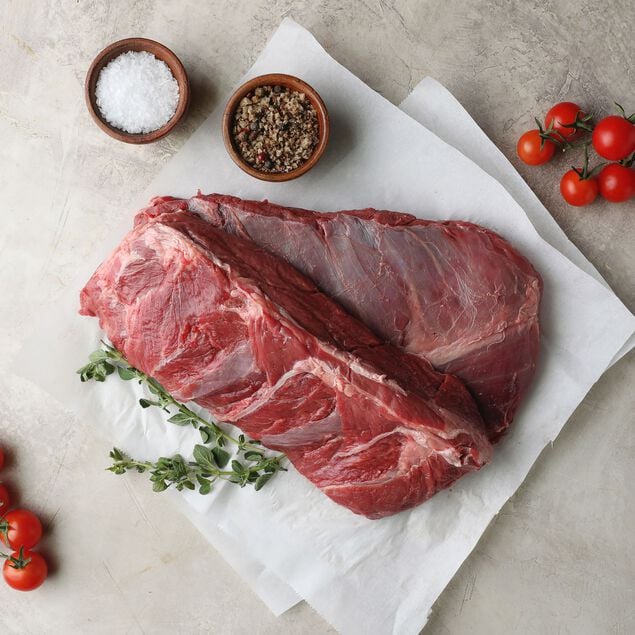In this image, we see two large, thick cuts of red, marbled beef sitting in the center, placed on a white butcher paper that is arranged in a diamond shape on an off-cream, granite countertop. Accompanying the meat, on the left side, there is a sprig of light green-gray thyme, while a couple of sprigs of parsley rest beside it. In the bottom left corner, a cluster of deep orange cherry tomatoes with green tops can be seen, and another similar cluster is present in the upper right. To the upper left of the beef are two medium brown wooden bowls, one filled with salt and the other with peppercorns. The scene is free of any text, making the rich colors and textures of the ingredients stand out vividly.